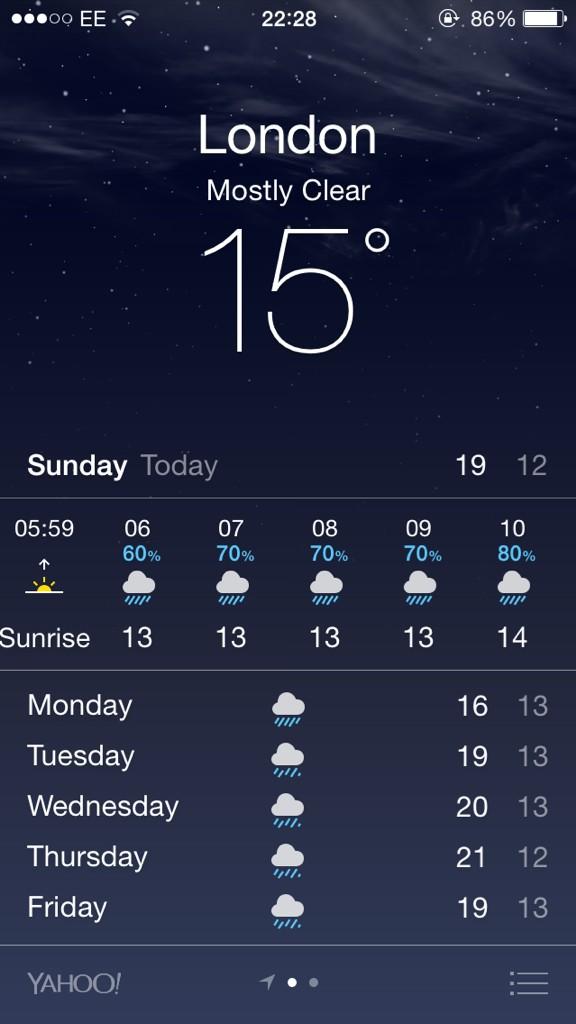The image depicts a dark blue night sky with scattered white stars and slightly visible white clouds. Displayed on a smartphone, this is a screenshot of a weather application. The time on the phone reads 22:28, indicating nighttime. The application’s text is white for clarity against the dark background.

At the center top, the weather forecast for London is prominently displayed. It reads: "London, mostly clear, 15°C." Below that, additional details for Sunday are provided: a high of 19°C and a low of 12°C. The hourly weather forecast starts from 05:59 with the sunrise and continues for each hour: 
- 6:00 - 13°C, 60% precipitation (percentages are written in blue),
- 7:00 - 13°C, 70% precipitation,
- 8:00 - 13°C, 70% precipitation,
- 9:00 - 13°C, 70% precipitation,
- 10:00 - 14°C, 80% precipitation.

Further down, the weekly forecast is shown:
- Monday: High of 16°C, Low of 13°C,
- Tuesday: High of 19°C, Low of 13°C,
- Wednesday: High of 20°C, Low of 13°C,
- Thursday: High of 21°C, Low of 12°C,
- Friday: High of 19°C, Low of 13°C.

At the bottom left corner, the word "Yahoo" is displayed, likely indicating the source of the weather data. In the bottom right corner, there is a menu icon for additional options.